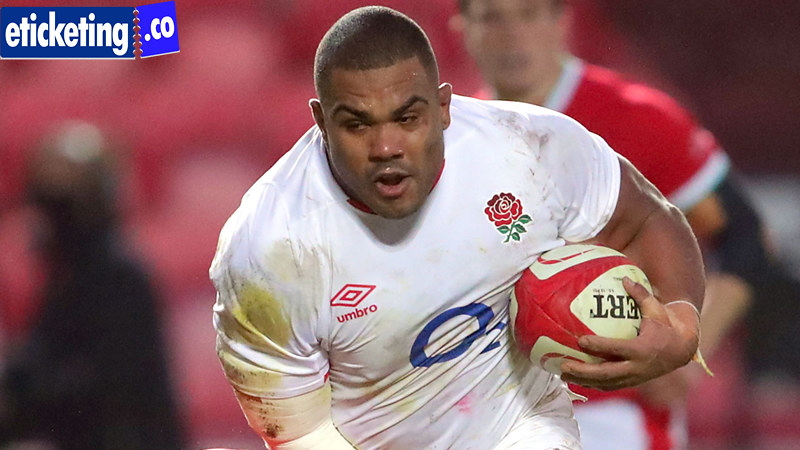The image captures a muscular soccer player with short black hair, hunched forward and to the left, wearing a sweat-stained white jersey marred by dirt and yellowish discoloration. His expression is intense and focused, with mouth open and eyebrows raised, framed by dark skin. Clutched under his right arm is a red and white ball adorned with black lettering. Centered on his chest is a blue circular emblem, while the upper right side of his chest features a red rose with green leaves beneath it, and the left side bears a red diamond containing a smaller diamond with "UMBRO" written in red below it. The upper left corner of his jersey displays a blue square inscribed with "E-TICKETING DOTCO." The background is notably blurry, yet discernible is a person standing behind him in a red shirt adorned with white accents around the sleeves and neck, and wearing a black elbow brace. The overall scene, shot from a low waist-level angle, emphasizes the player's gritty determination amidst the action.